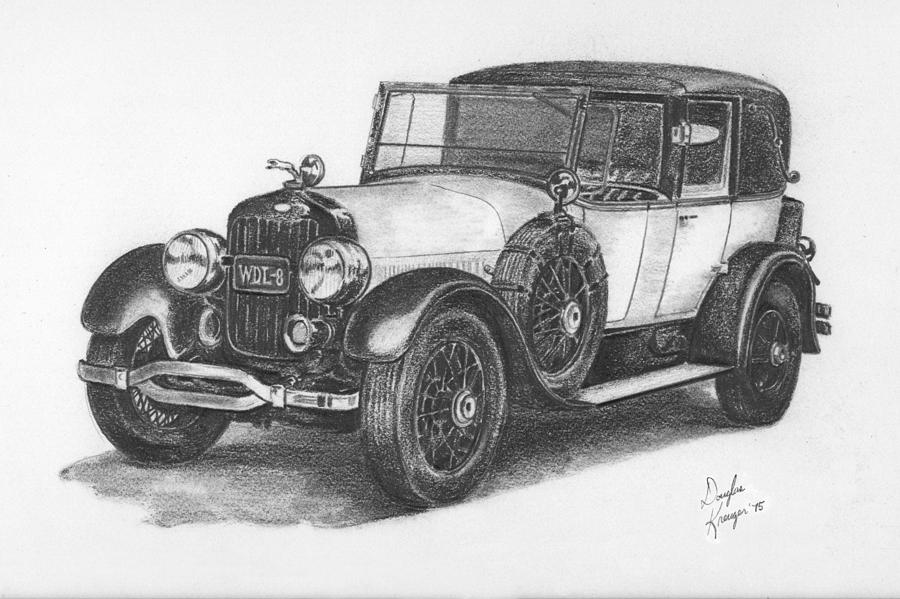The detailed sketch, signed "Douglas Kruger, 75" in the bottom right corner, features a meticulously drawn vintage car set against a soft grey background. This black-and-white pencil drawing showcases an old-fashioned, two-door vehicle with a backseat. The car occupies the right side of the image, with its rounded top and extended hood facing left. Notable details include a black hood adorned with an ornament that resembles either a bird or a snake's head, and a prominently placed rectangular windshield. The car sports skinny wheels with spoke rims, including a spare wheel mounted on the driver's side of the hood. Its front grille is black with silver accents and houses a rectangular license plate marked "WDL8," situated between two perfectly round, spotlight-like headlights.